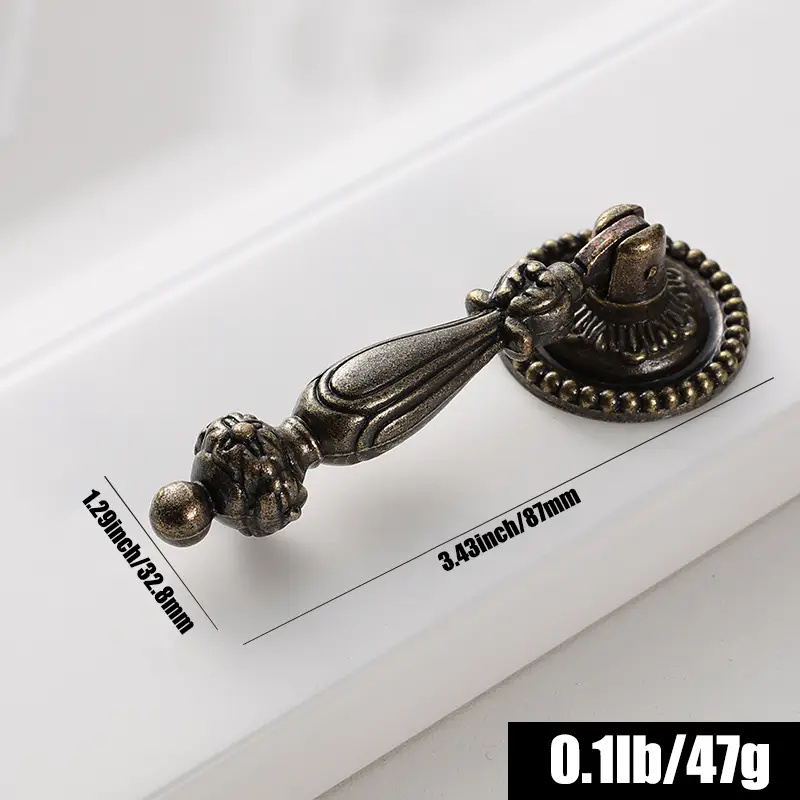This detailed color photograph, likely taken indoors with artificial lighting, features a shiny, elaborate bronze doorknob installed on a white door. The composition is slightly diagonal, orienting the knob from the bottom left to the top right. The knob itself has a sculpted handle and a tapered body leading to a circular base where it attaches to the door. The circle is adorned with a delicate bead-like pattern along its circumference. Additionally, the image includes precise measurements in black text along the top and bottom of the knob: “1.29 inches / 32.8 millimeters” and “3.43 inches / 87 millimeters,” respectively. In the bottom right corner, within a black rectangular box, white text displays the weight of the knob: “0.1 pounds / 47 grams.” The overall setting appears professionally staged, possibly with digital enhancements to highlight the product's details.